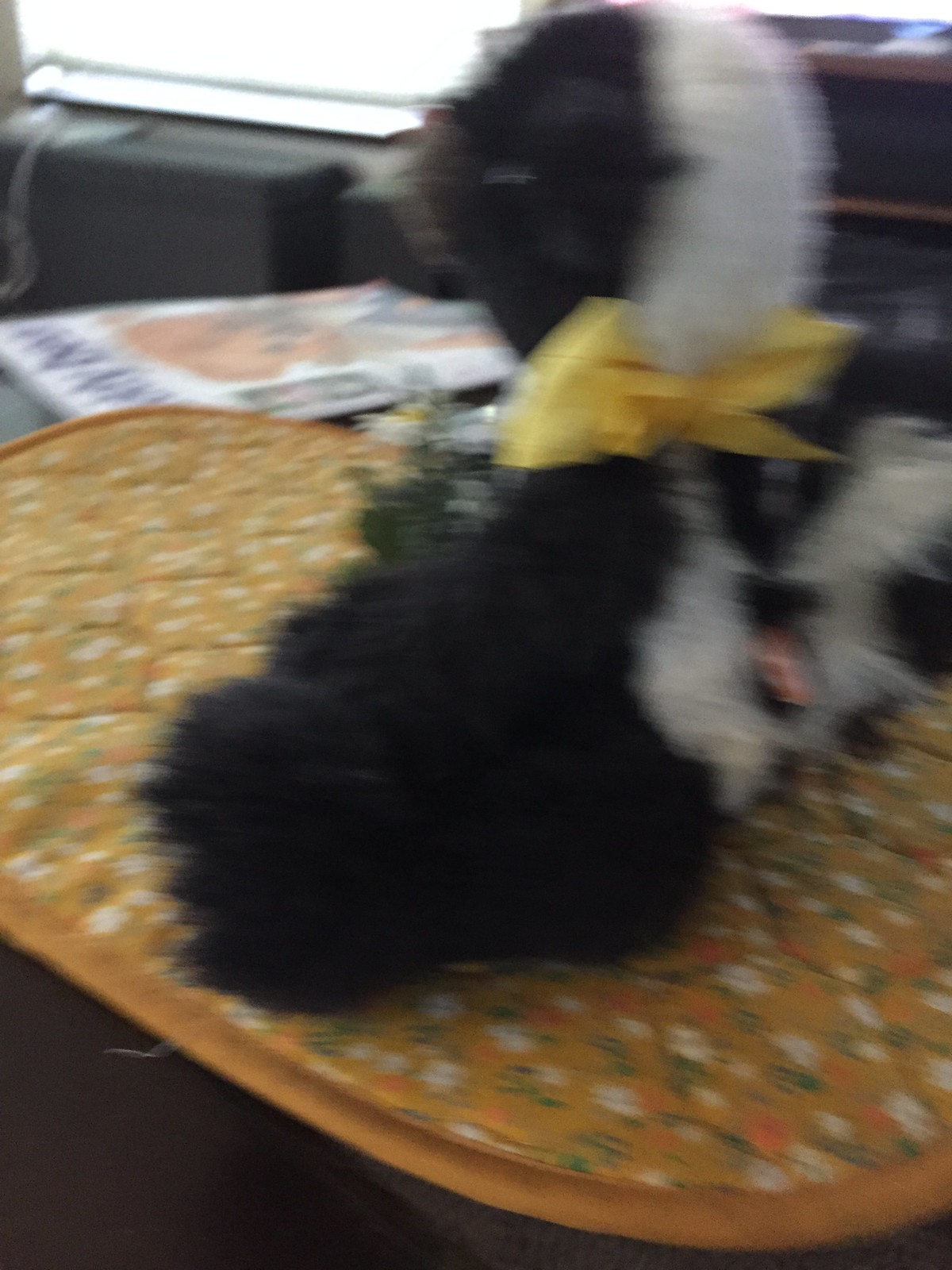The photo shows a blurry, out-of-focus interior of a house, with a polished, dark brown-reddish wooden table at the center. On the table lies a fabric placemat with a green and white paisley pattern, interspersed with white and orange flowers and green stems. Atop this placemat is a black and white stuffed animal, possibly a skunk given its black eye and yellow bow around its neck. There is some ambiguity due to the blurriness, but it could also be a teddy bear-like toy. In the background, you can discern a flat-screen TV or window streaming sunlight, along with a magazine featuring a picture of a teddy bear, resting on the same table.